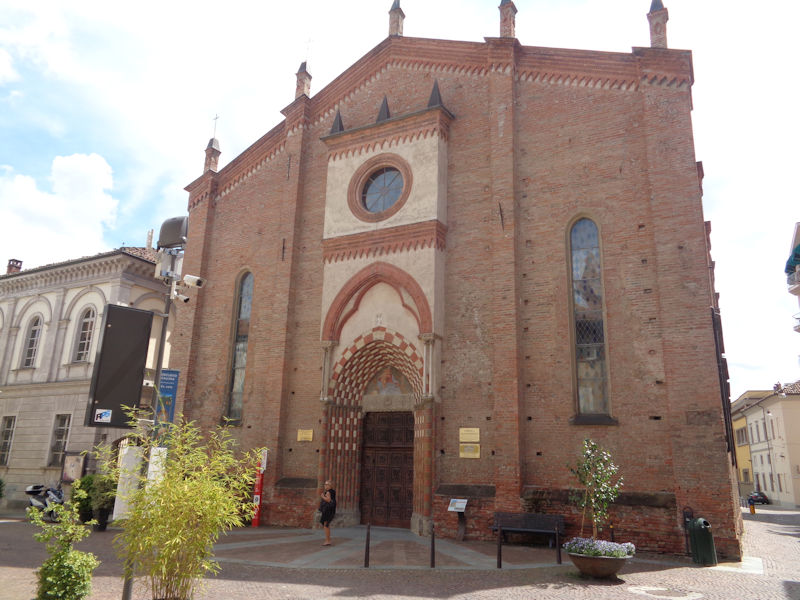The image shows a tall church situated on a street corner, constructed with a dark brown brick facade that adds to its historic appearance. The church features an angled roof with spire-like columns, one of which prominently displays a cross. The front of the church is adorned with several oval-shaped stained glass windows, including two long thin ones on either side of a striking circular window positioned at the center top. Below this circular window, additional brick embellishments enhance the facade. There's a large archway above the main entrance, which consists of dark brown wooden double doors framed by terracotta and beige stonework, adding layers and depth to the design.

In front of the church stands a Caucasian woman dressed in a black sleeveless shirt and black skirt. Her blonde hair stands out against the backdrop. Surrounding her are various elements that add to the building's detailed environment: a small decorative plant in a pot, a black table, and a round brown trash can. There’s also a black trash can to the right of the building, placed near a table and a purple-flowered plant. Additionally, two small circular video cameras are mounted on the left side of the building for security.

Three gold plaques are attached to the front of the church—one on the left side of the door and two on the right—adding to its historical significance. There's also a standing plaque in front of the church. A bench is placed to the right side of the building. The image captures some of the surrounding area, including a partial view of a gray building to the left and a yellow and white building down an alleyway on the right. The sky overhead is blue with scattered white clouds, adding a serene backdrop to this detailed scene.